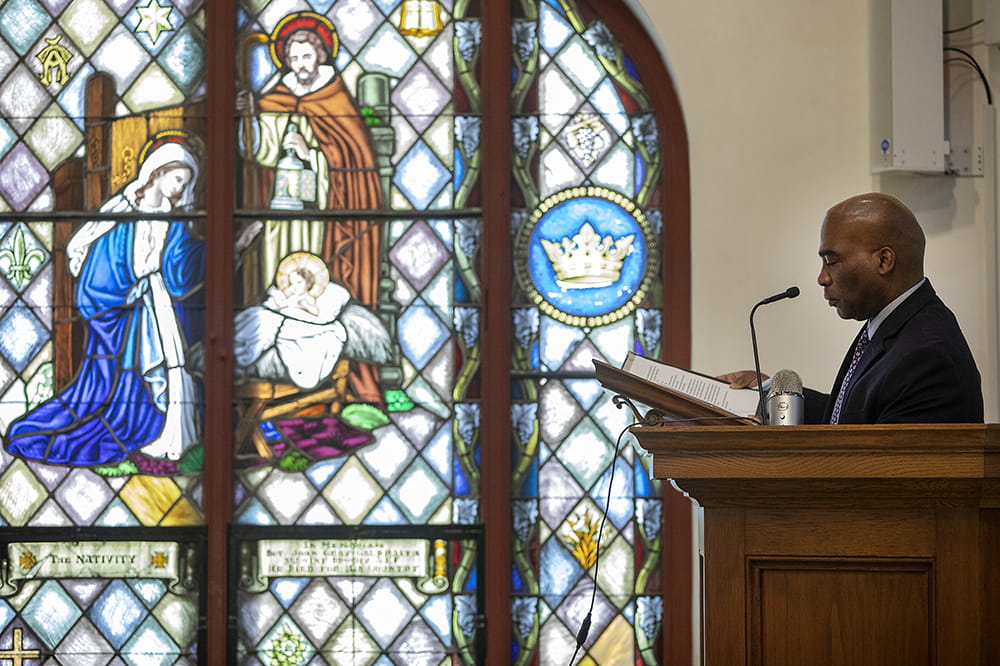The image is a color photograph captured inside a church, presented in a landscape layout. In the center of the frame, a bald man, viewed from the side, stands at a brown wooden pulpit, reading from a large book. He is dressed in a dark jacket with a collared white shirt and a tie. Positioned in front of him is a small microphone just above his mouth. The wall behind him is white, featuring a speaker above his head. Dominating the background is a large, arched stained glass window framed in brown wood. The stained glass portrays the nativity scene with Mary, Joseph, and the baby Jesus lying in a manger, surrounded by colorful cloths. The intricate design consists of diamond patterns in various hues of blue, along with accents of oranges, browns, yellows, greens, and purples. Within the blue segment of the stained glass, there is a circular motif rimmed in gold, showcasing a crown inside. The setting appears serene, focused solely on the preacher as he delivers his sermon.